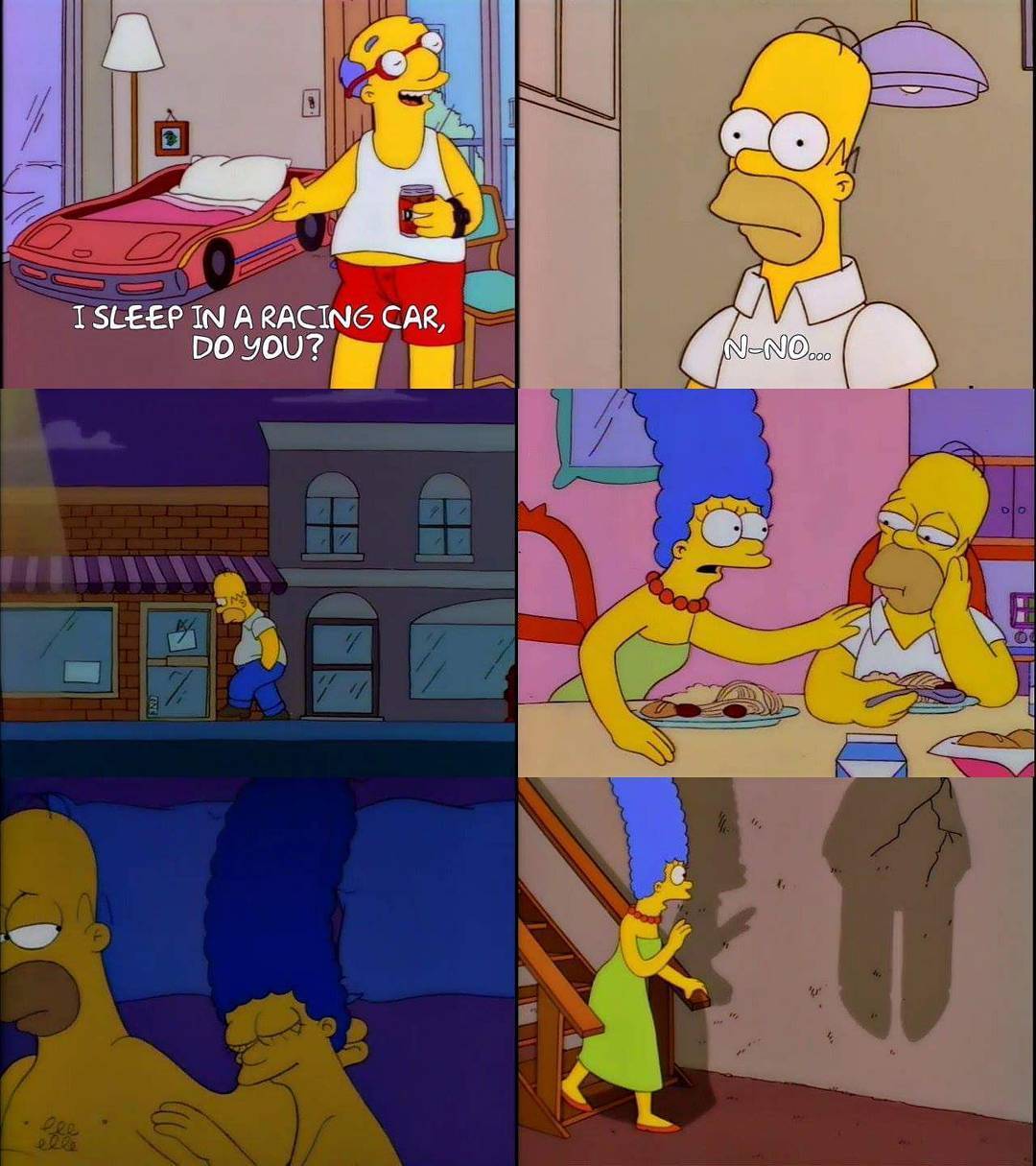The image is a detailed comic strip from The Simpsons, comprising six scenes presented in a grid. In the top-left scene, Grandpa Simpson stands in a child's bedroom featuring a red race car bed with a white pillow and pink blanket. He is casually dressed in a tank top and red boxers, holding a drink, with an open window covered by an orange curtain behind him. The caption reads, "I sleep in a racing car, do you?" To the right, Homer Simpson, wearing an off-white shirt with the letters "N-N-O..." printed below it, responds simply with, "No."

The middle-left scene shows Homer walking down the street at night, hands in his pockets and head down, looking contemplative. He wears blue pants and a grayish-green shirt. The middle-right scene depicts Homer and Marge at the dinner table. Marge is leaning towards Homer with her hand on his shoulder, while Homer, holding a spoon, looks either at her or down at his plate.

In the bottom-left scene, Homer and Marge are in bed. Marge, eyes closed, rests her head on Homer's arm, while Homer gazes at her. They are covered with a purple blanket and rest on blue pillows. The bottom-right scene shows Marge descending a staircase, wearing a green dress, red pearls, and red slippers. She gasps in shock at a shadow on the wall, which appears to depict a figure hanging, adding an eerie twist to the otherwise domestic scenes.